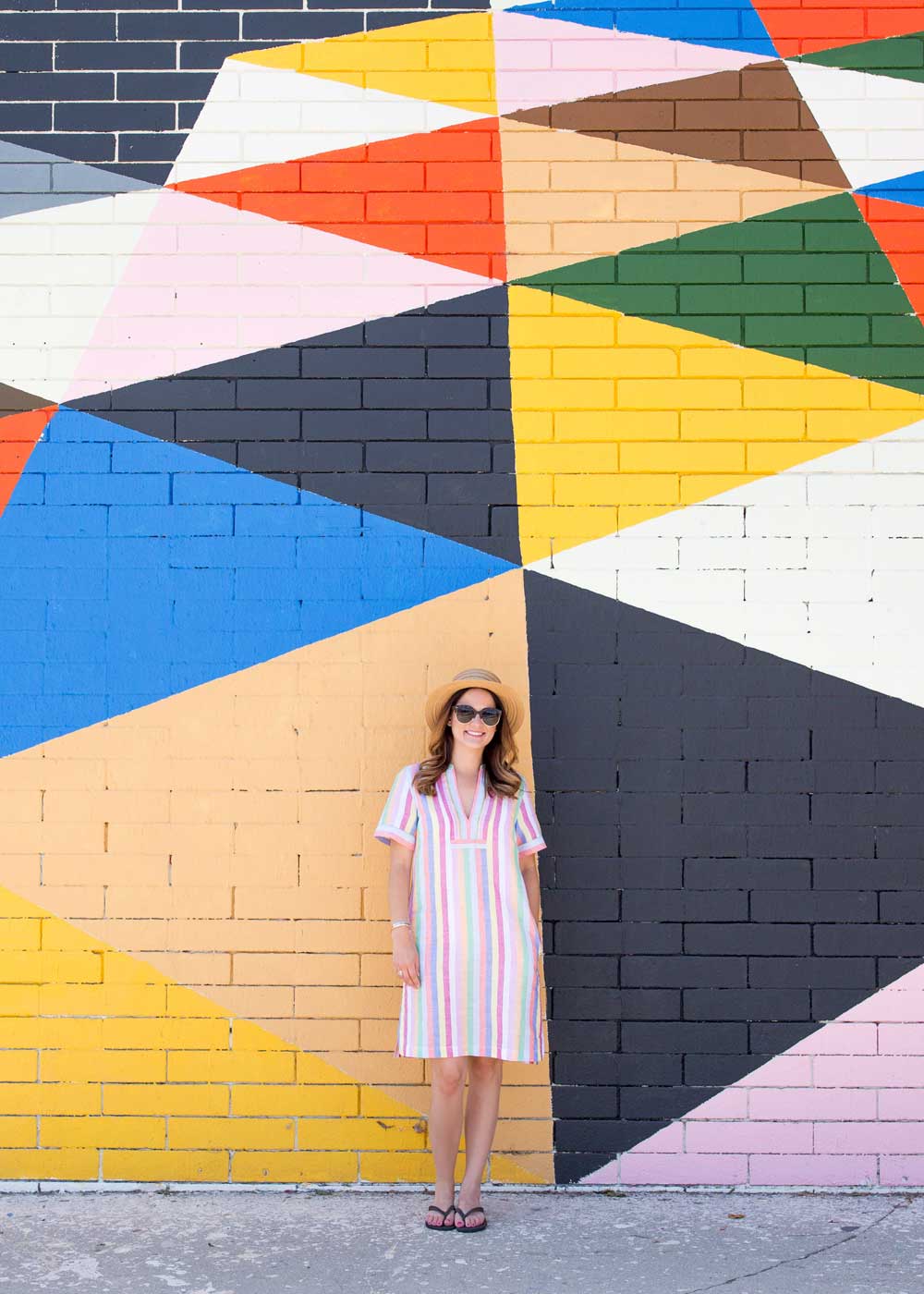In this photograph, a woman stands confidently, posing in front of a vibrant, geometric mural on a brick wall. The mural features an array of colorful, triangular patterns in shades of blue, black, yellow, green, orange, white, pink, and occasionally brown, with some sections of the brick wall left unpainted at the top left corner. The woman is centered at the bottom of the image, standing on a gray pavement. She is dressed in a knee-length, light-colored striped dress, with hues of white, pink, blue, and green, contributing to the summery vibe. She accessorizes with a wide-brimmed hat, sunglasses, and black flip-flop sandals. She has shoulder-length hair and is smiling warmly at the camera, adding a lively human element to the bold graphic background. The photograph captures a striking contrast between her summery appearance and the dynamic, painted triangles of the mural behind her.